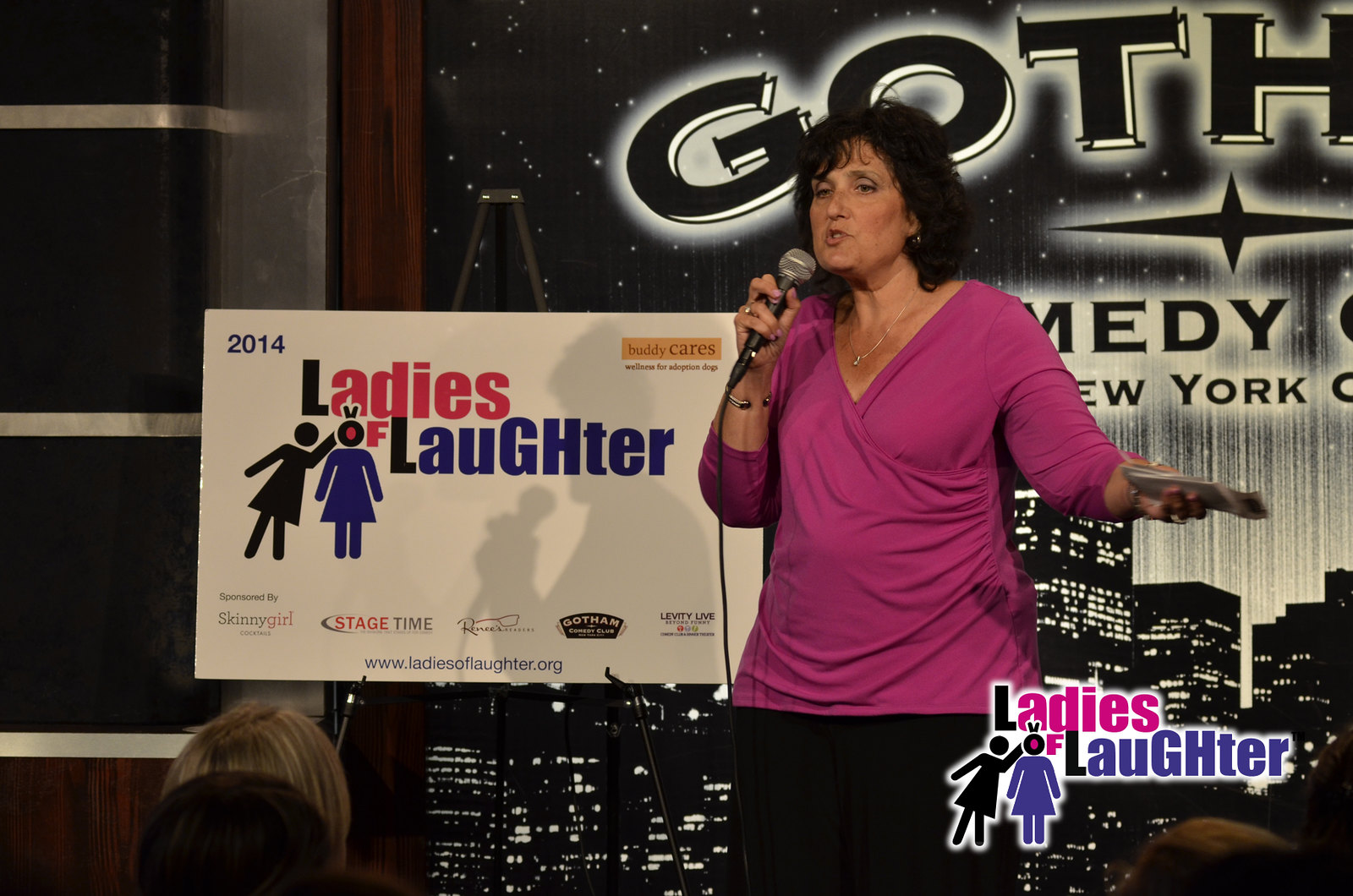This photograph captures a woman performing a comedy routine at the renowned Gotham Comedy Club in New York City, as indicated by the partially visible club name in the background. She is the focal point, standing confidently on stage wearing a vibrant magenta v-neck tunic paired with a gold necklace, a ring, and an elegant bracelet that doesn't close entirely. Her shoulder-length, slightly curly hair frames her expressive face. She holds a microphone in her right hand and note cards, possibly cue cards, in her left.

The stage backdrop is adorned with signage for the "Ladies of Laughter" event, displayed prominently in a mix of black, magenta, and purple fonts. The signage includes various sponsors, such as Skinny Girl Cocktails, Stage Time, Gotham Comedy Club, and Levity Live, along with a website URL ladiesoflaughter.org. It also features a cardboard placard with two female figures and identifies the year 2014. This detailed scene encapsulates the vibrant atmosphere of a comedy performance dedicated to showcasing female comedians.